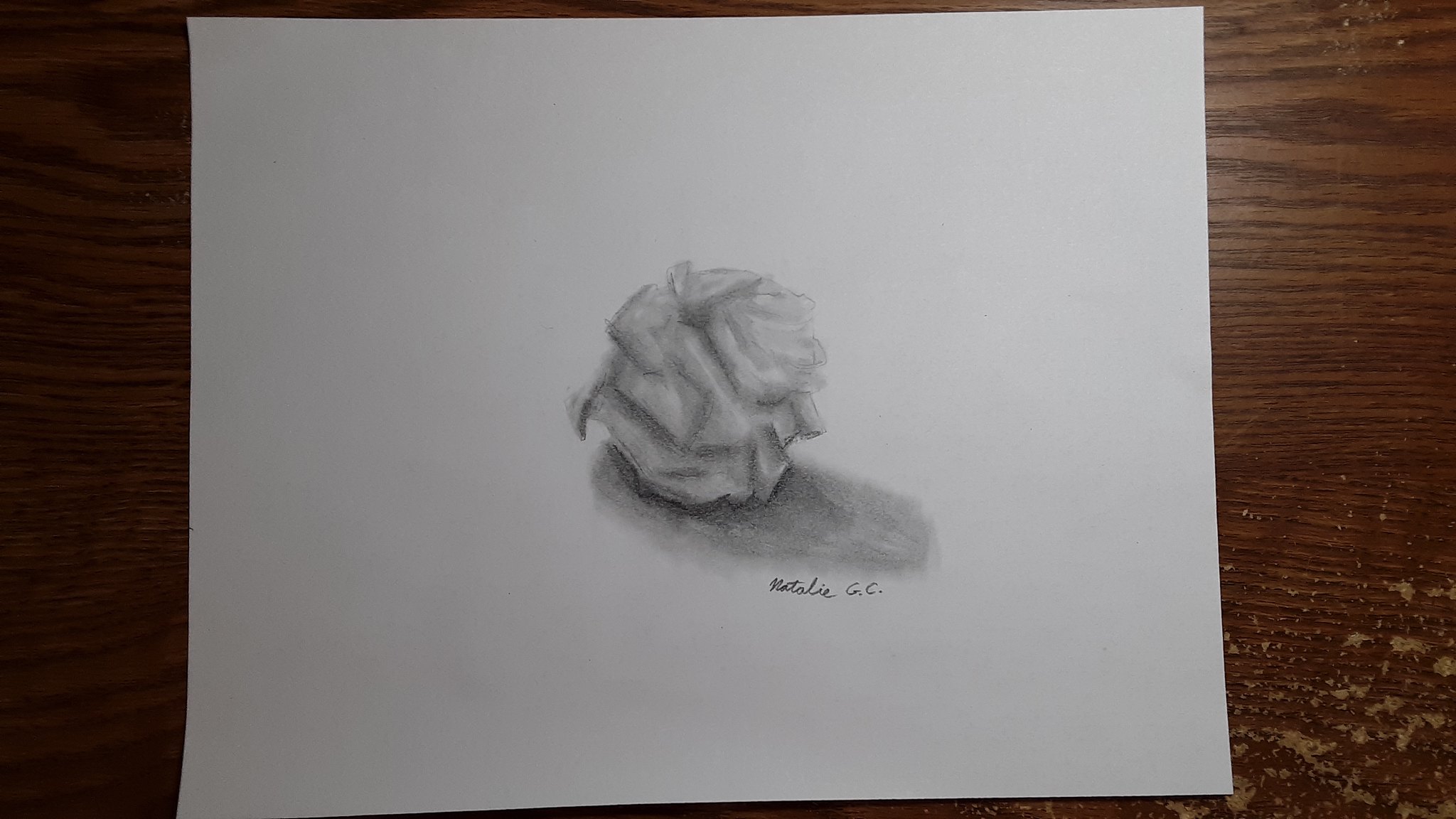The image captures a large piece of white sketch paper centered on a mahogany table, featuring distinct wood grain patterns in both dark and light shades. The table's well-used condition is highlighted by visible imperfections such as scuffs and possible water damage with bubbled and peeling areas, especially noticeable in the bottom right corner. In the middle of the sketch paper, there is a faint, grayscale pencil drawing of what appears to be a crumpled ball of paper. The drawing incorporates detailed shading and folds, complete with a shadow beneath it, indicating a light source from the upper left side. The bottom of the drawing bears the artist's signature, "Natalie GC." Despite the careful attention to shadows and highlights, the overall execution of the drawing appears somewhat lacking in precision. The photograph of the scene is taken from a distance, showing most of the paper and just the edges of the table. The lighting in the photograph itself seems to come from the upper right.